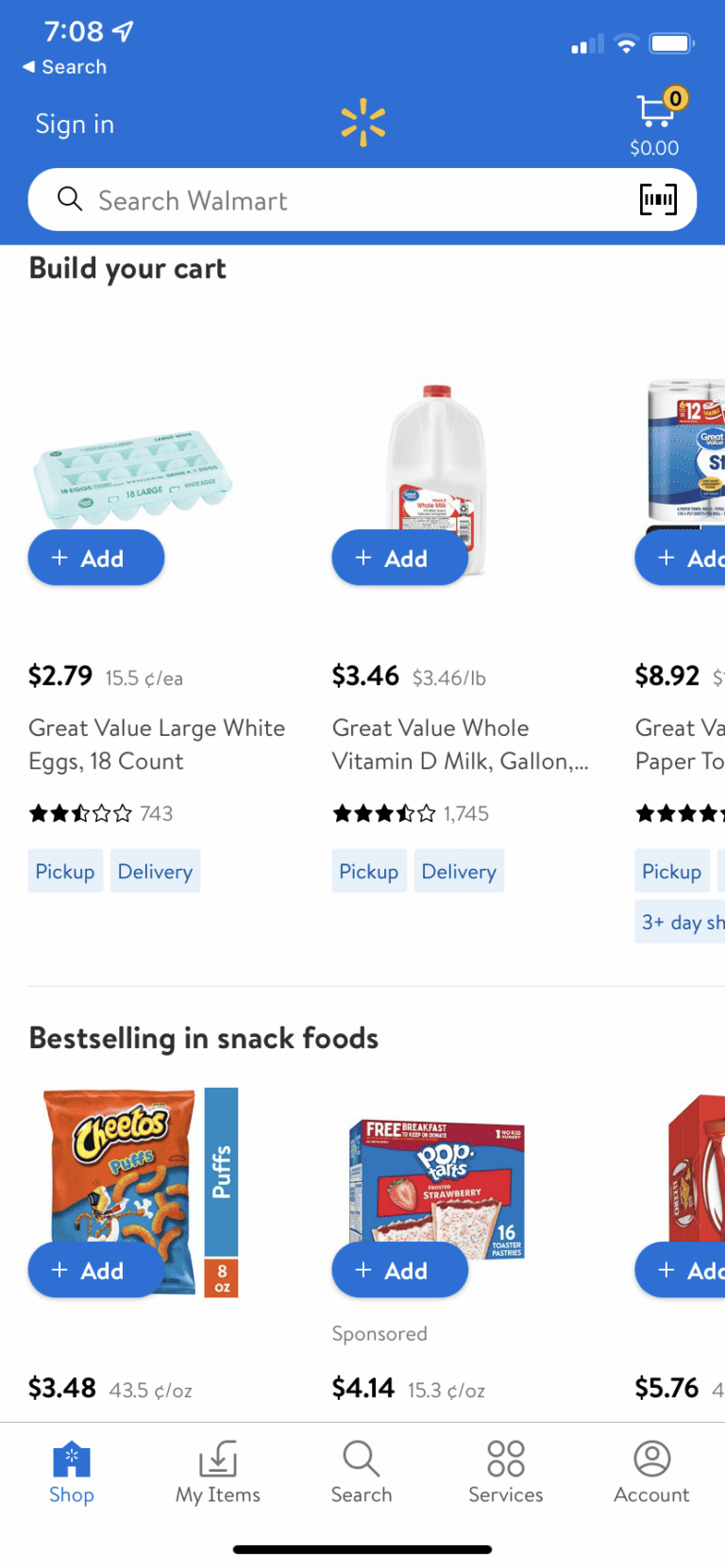Screenshot of the Walmart App Interface

In this detailed screenshot of the Walmart app, the time is displayed in the top left corner at 7:08 a.m. Nearby, a navigational arrow is visible alongside indicators showing 3 bars of cellular signal strength, 2 bars of Wi-Fi signal, and a fully charged battery. Directly below the time, there is a back arrow and a prominent search button. Beneath this, users will find the "Sign In" button.

At the center of the screen, the iconic Walmart logo—a yellow sunburst—stands out. To the right of the logo, there is a shopping cart icon currently showing zero items. A white search bar, prompting users to "Search Walmart," sits just below the logo, accompanied by a barcode icon to facilitate scanning items for search.

The app encourages users to "Build Your Cart" as highlighted at the top of the screen. The detailed product listings include:

- Great Value Large White Eggs (18 count) for $2.79
- Great Value Whole Vitamin D Milk (gallon) for $3.46
- Great Value Paper Towels for $8.92

The "Best Selling in Snack Foods" section features popular items such as:

- Cheetos Puffs for $3.48
- Strawberry flavored Pop-Tarts (box) for $4.14
- Cheez-Its Snack Bags (box) for $5.76

This screenshot showcases the intuitive layout and functionality of the Walmart app, designed to streamline the shopping experience.